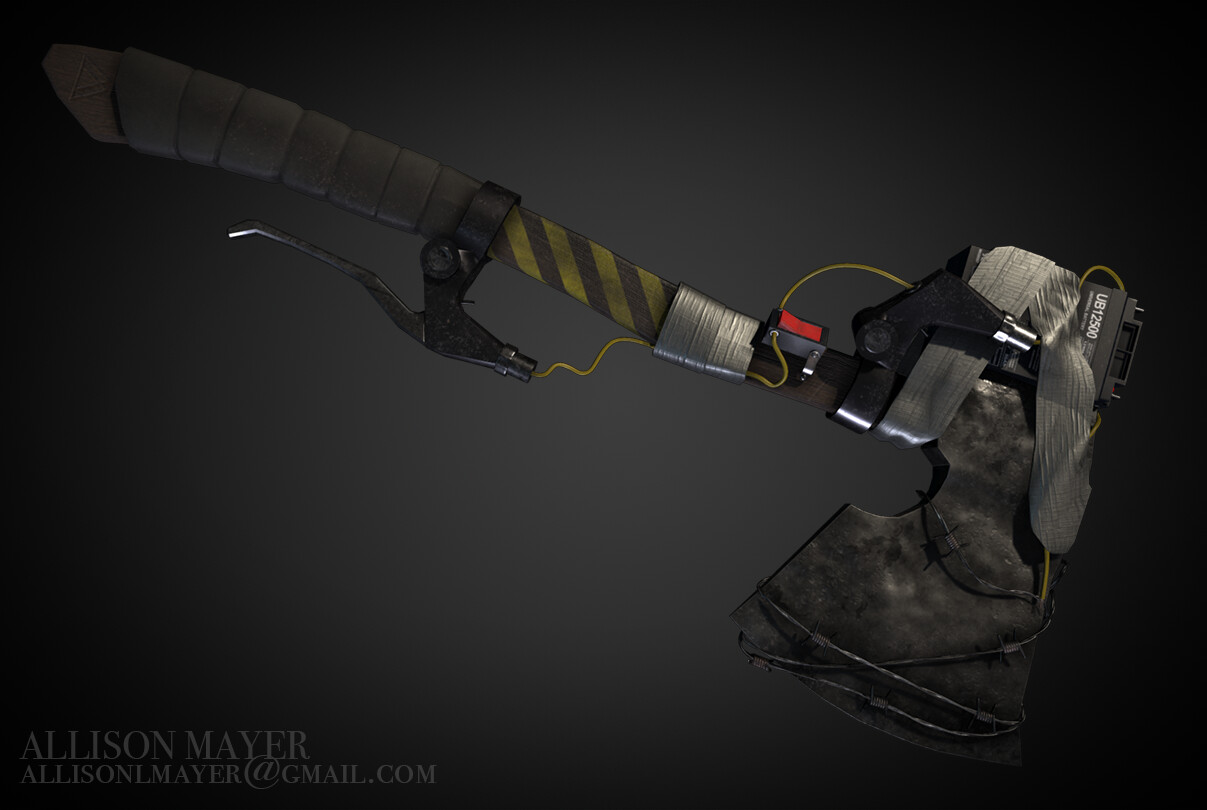The image depicts an artist's rendering of an inventive makeshift automatic axe, bearing distinctive characteristics of a traditional axe with added complex machinery. The axe features a black handle, potentially made from rubber or styrofoam, for a firm grip. A prominent detail is the yellow and black striped pattern in the center, likely indicating a cautionary or operative component. Integrated into the handle is a trigger mechanism resembling a bicycle brake handle, designed to activate the axe head, suggesting movement or an automated chopping function possibly powered by an attached battery or chip. Yellow wires extend from the trigger up to an articulating joint and are connected to additional machinery near the axe's head, which includes what appears to be a battery labeled "UB12500" or "LB12500" and an indiscernible text. The axe head itself is black with elements of mottled gray and encircled by metal wire, giving it a rugged appearance reinforced with bandages or duct tape, signifying its makeshift origin. This complex and imaginative design is set against a stark black background that transitions from a bright center to darker edges, presenting a dramatic focus on the axe. At the lower left corner, the image credits the artist, Allison Mayer, with her email address, allisonmayer@gmail.com, in light gray lettering.